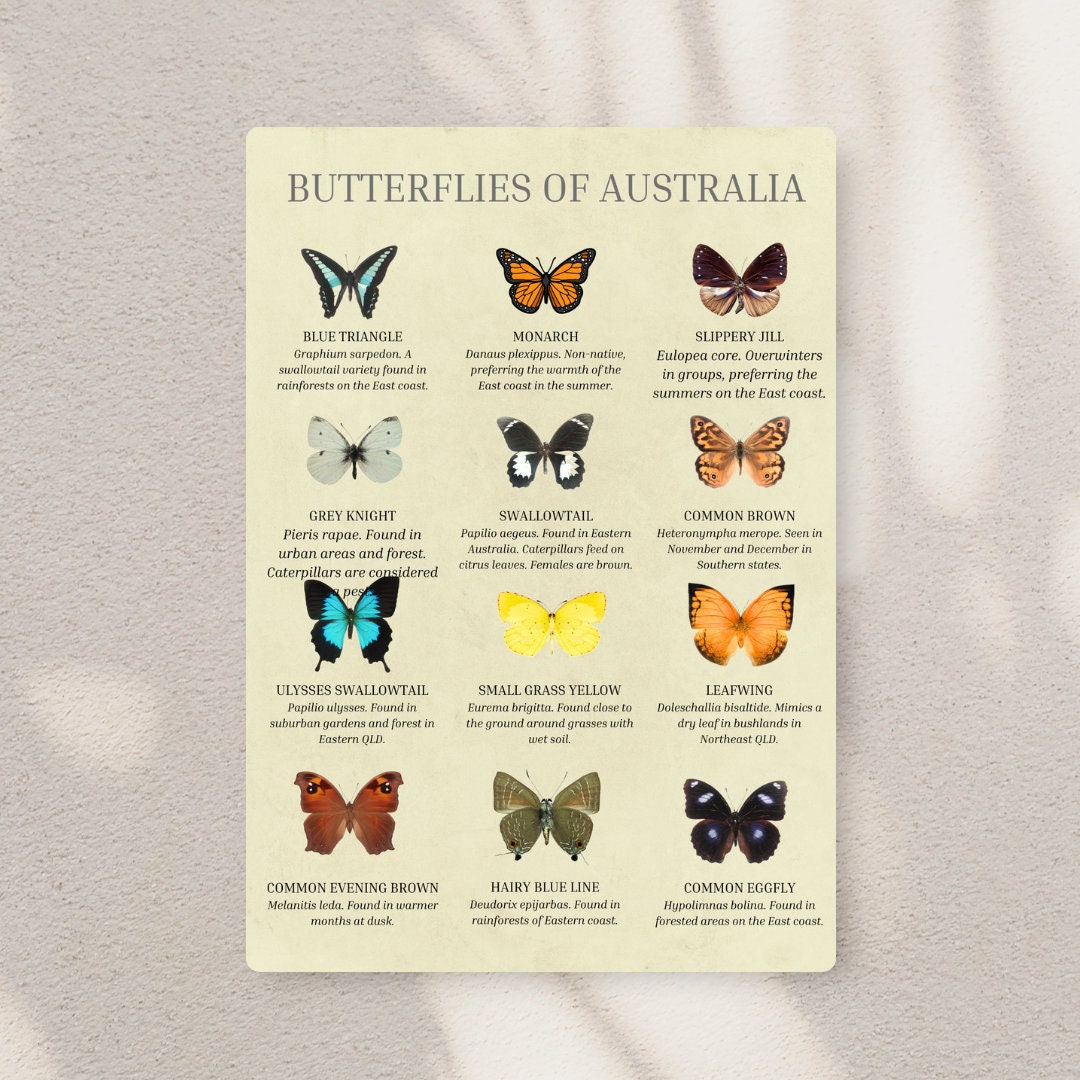The photograph captures a poster titled "Butterflies of Australia," set against a pristine white background illuminated by natural sunlight, creating subtle white spots on the backdrop. The poster occupies approximately 45-50% of the image and features a collection of 12 butterflies, meticulously illustrated with their wings fully spread. These butterflies are arranged neatly in three columns and four rows, with each species’ name inscribed beneath its respective image. The background of the poster itself is a very light yellow, enhancing the vivid array of colors displayed by the butterflies.

From left to right and top to bottom, the butterflies are: the Blue Triangle, with its iconic blue and black outline; the Monarch, known for its black-outlined orange compartmentalized pattern; the Slippery Jill, which transitions from dark purple at the top to a lighter white towards the bottom of its wings; the purely white Gray Knight with a black body; the Swallowtail, which is predominantly black with small white-spiked circles on the lower wings; the earthy-toned Common Brown; the Ulysses Swallowtail, showcasing a vibrant oceanic blue within its black outlines; the purely yellow Small Grass Yellow; the bright orange Leafwing with a subtle black outline; the leafy brown Common Evening Brown, distinguished by two black dots on its upper wings; the dull gray, faintly blue-bodied Hairy Blue Line; and the Common Eggfly, characterized by its predominantly black wings adorned with dark purple and distinctive white patches.

Each butterfly is not only named but also accompanied by a brief description below its image, making this poster both visually captivating and educational.